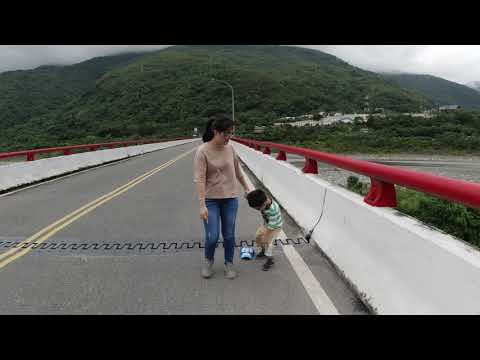In this photorealistic image of a poor resolution photograph, a woman with dark hair in a ponytail and glasses stands on a long bridge, holding the hand of a small child. She is wearing a light brown long-sleeve shirt, blue jeans, and gray shoes. The child beside her, possibly her son, has black hair and wears a green and white striped shirt, khaki-colored pants, and black shoes. The child appears to be looking down at a blue and white hat that has fallen to the ground.

The bridge features white barriers with a red metal fencing on top, positioned along both sides. The road on the bridge, gray in color, has a double yellow line running down the center and a noticeable zigzag line crossing from left to right. To the right side of the bridge, an area void of trees and appearing gray in color suggests a body of water, indicating that the bridge spans a river. Small white buildings are visible to the right in the distance. Beyond the bridge, large, rolling hills or mountainous areas are covered in dense dark green foliage. Above these hills, dense white areas, possibly clouds, sky, or fog, cap the horizon, completing the scene.